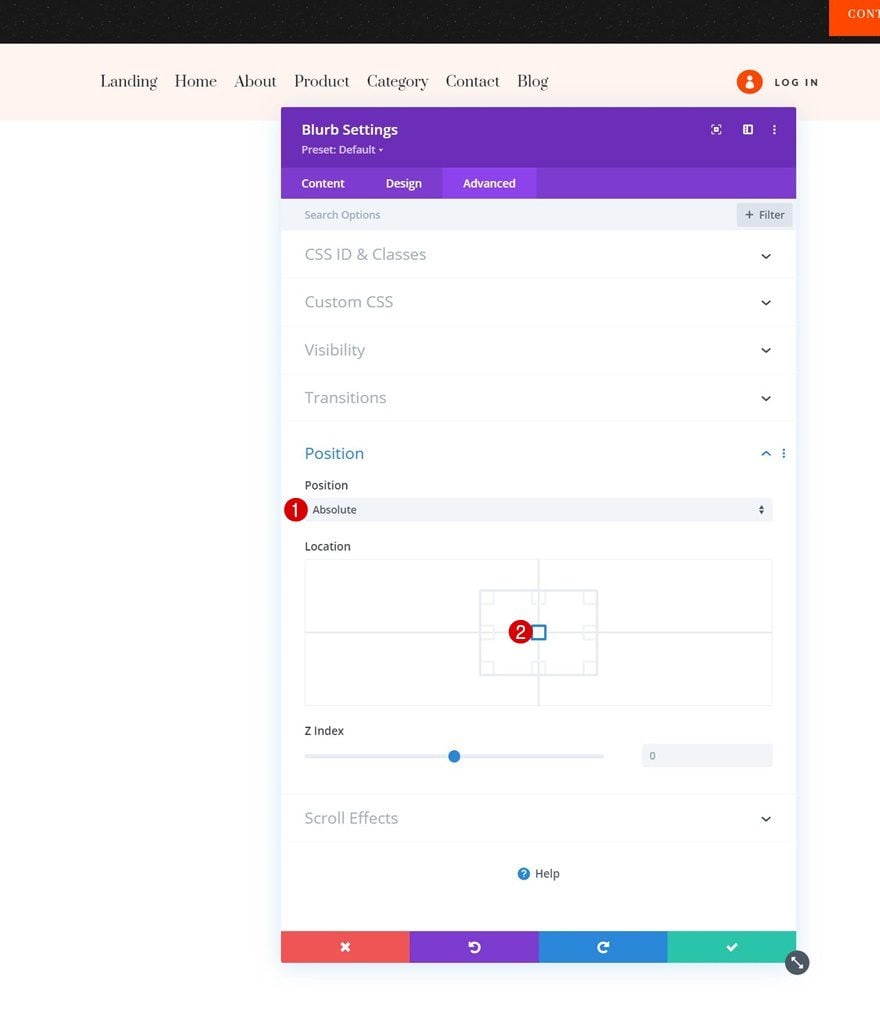The image depicts a detailed layout of a website interface. At the top, it features a navigation bar with clickable tabs labeled, from left to right, as Landing, Home, About, Product, Category, Contact, and Blog, accompanied by a login button on the right. 

Centrally located is a section titled "Blurb Settings" with configurations set to Preset: Default. Beneath this, there are three sections: Content, Design, and Advanced. 

The Advanced section is further divided into specific options: CSS ID & Classes, Custom CSS, Visibility, and Transitions. Each of these options is presented in a row format. Below these rows is a section labeled "Position" which is expanded to display 'Absolute' positioning. 

Additionally, there is a visual representation involving a square box within another box, numbered '2' in red, slightly off-center to the left. Adjacent to this, the Z-Index setting can be adjusted via a movable dot dial. Sound effects options are also available below this section. 

The interface provides various control buttons at the bottom: a red X to close the settings, a purple left-pointing arrow to go back, a blue right-pointing arrow to move forward, and a green check mark to confirm changes.